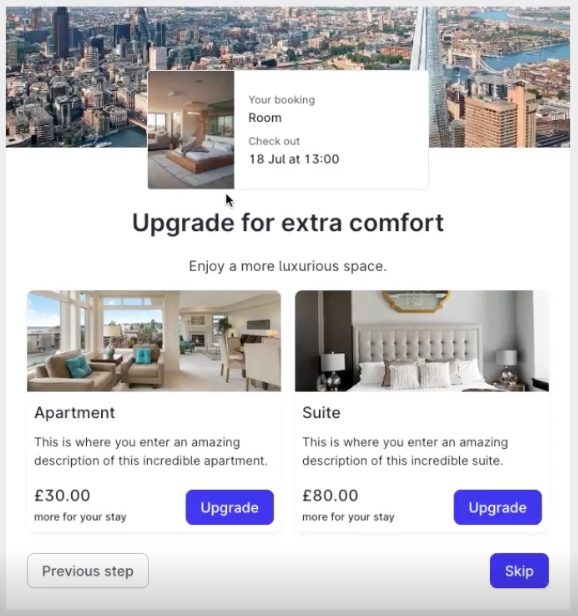The screenshot displays a website offering bookings for both apartments and suites, resembling a hybrid of an Airbnb and a hotel service. The website's layout includes a top section confirming the user's booking details, indicating a room reservation with checkout scheduled for July 18th at 1:00 PM. 

At the bottom of the page, two options are presented for upgrading the stay: "Apartment" on the left and "Suite" on the right. The descriptions for both options are placeholders, reading "This is where you enter an amazing description of this incredible apartment" and "This is where you enter a basic description of this incredible suite," respectively.

- **Apartment Upgrade:** This option costs an additional 30 pounds and promises extra comfort for a more luxurious stay. A purple "Upgrade" button is available for selection.

- **Suite Upgrade:** Priced at 80 pounds more, the suite represents a higher-end option. It also features a purple "Upgrade" button.

Additionally, a promotional banner at the bottom encourages upgrading for superior comfort, enhancing the overall experience.